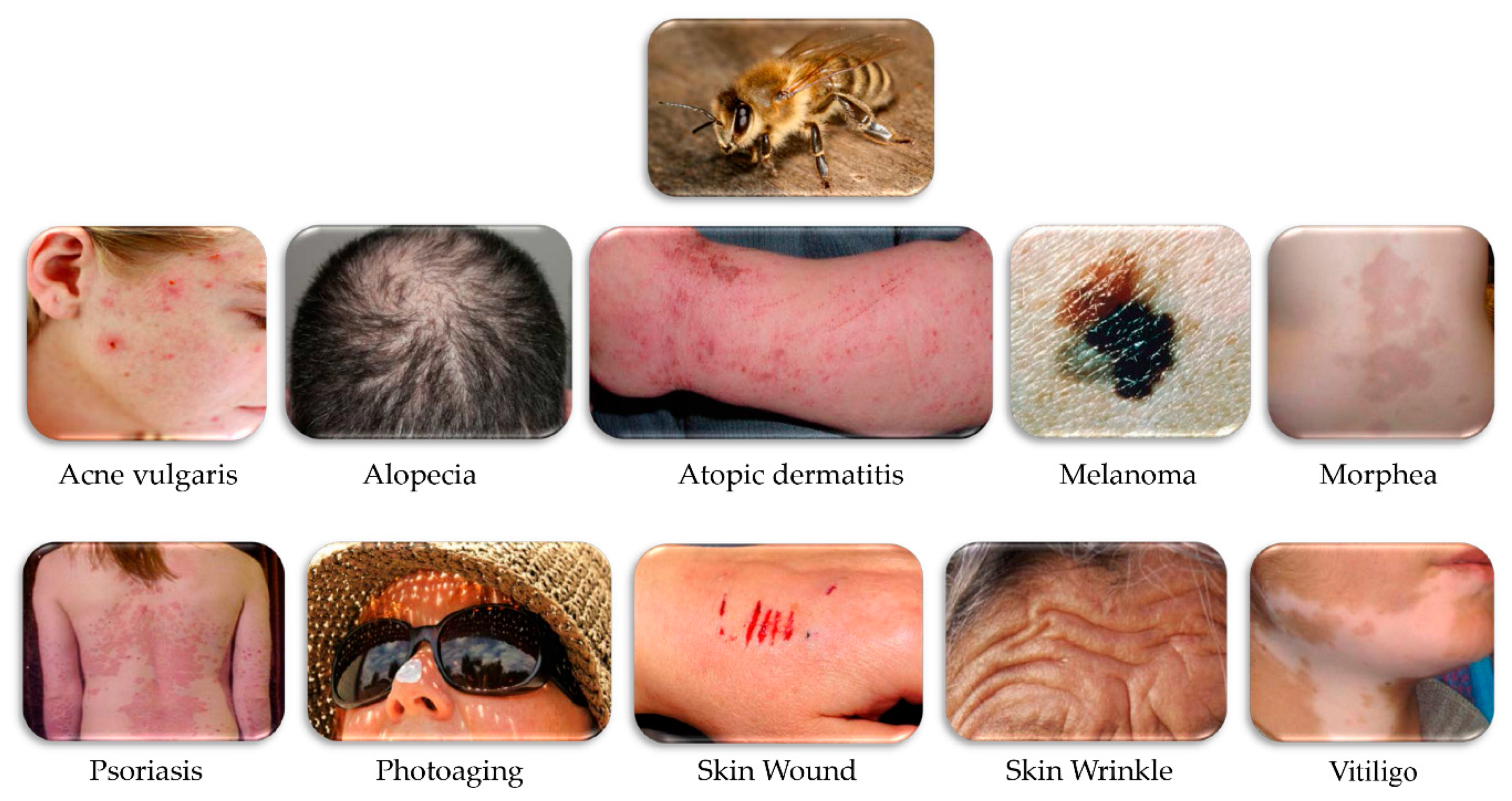The image features a detailed chart showcasing various skin conditions, all set against a white background. At the very top of the chart is a close-up photo of a bee. Below this, there are two rows each containing five color photos depicting different skin ailments. The top row, from left to right, includes photos labelled as acne vulgaris, alopecia, atopic dermatitis, melanoma, and morphia. In the bottom row, also from left to right, are photos labelled as psoriasis, photoaging, skin wound, skin wrinkles, and vitiligo. Each photo provides a clear, color depiction of the specific condition on actual human skin. The inclusion of the bee at the top is curious and its connection to the skin conditions shown in the chart is not immediately clear.